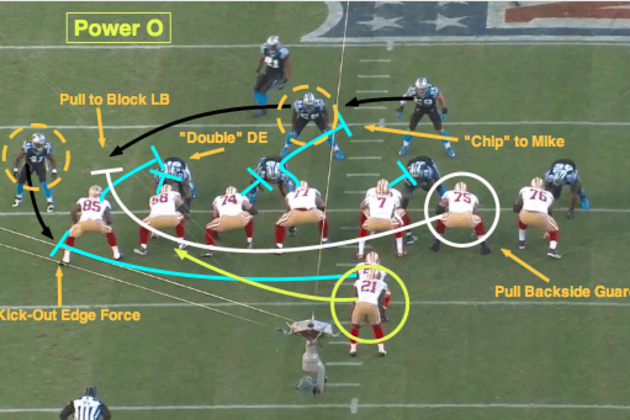The image is a detailed diagram of a football play, viewed from above, depicting a scene from what looks to be a video game. The field is comprised of short green grass with white yard lines, hash marks, and horizontal lines marking five-yard intervals. The NFL logo is partially visible at the top right corner. Players are positioned on the field, with one team likely resembling the San Francisco 49ers in white uniforms with red numbers, gold pants, and red socks. The opposing team, possibly the Carolina Panthers, appears in blue uniforms. The diagram features colored lines and arrows illustrating player movements and assignments, such as "pull to block LB," "double DE," "chip to Mike," "pull backside guard," "kick out edge force," and a play labeled "power O." The play's setup involves five players squatted down facing the opposing team, three more behind them, and detailed instructions for each player's actions during the play.